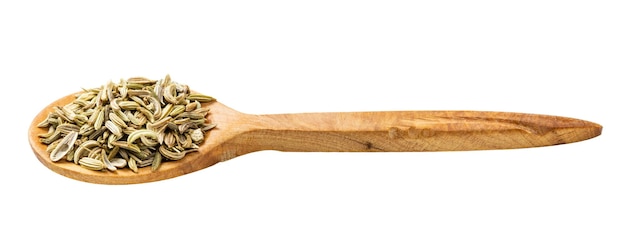The image shows a light-colored wooden spoon with a tan, marbled texture, lying flat on a plain white background. The handle, which is somewhat thick and pointed to the right, displays some darker brown marbling near the top. Inside the bowl of the spoon is an herb that appears to be rosemary. The small, greenish-whitish leaves of the herb are scattered in the spoon, resembling a bunch of tiny seeds or curled-up leaves.